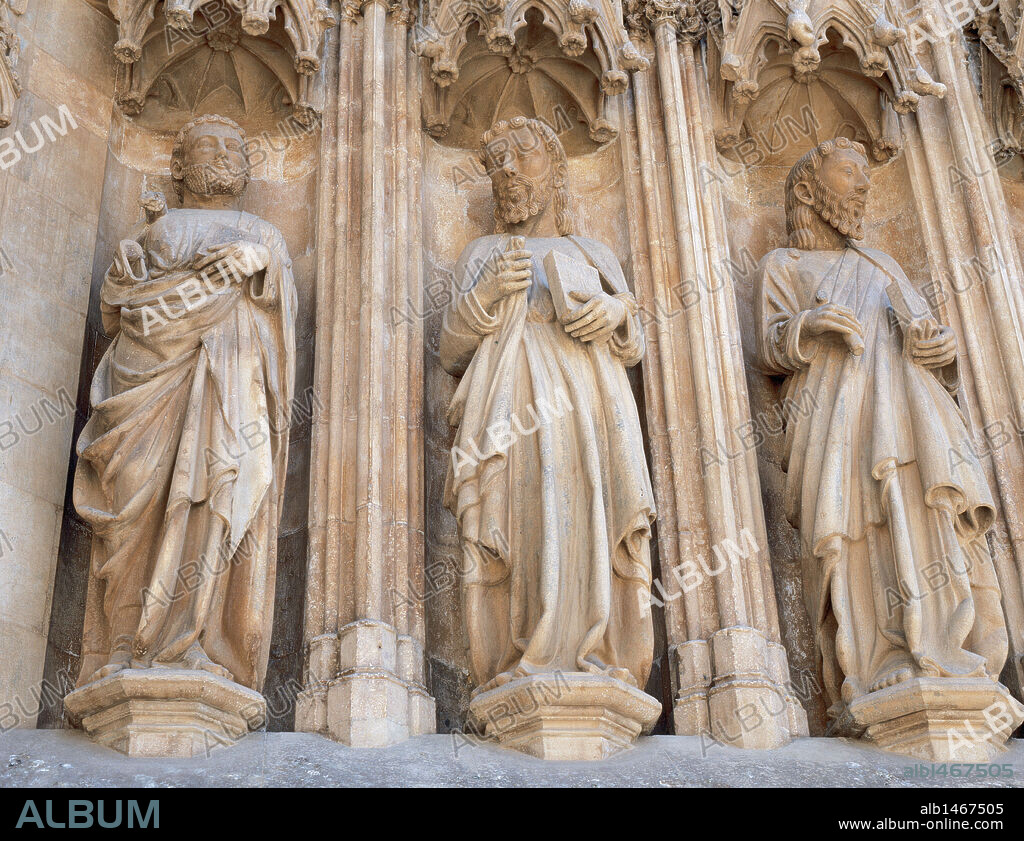This photograph, intended to be used for educational purposes or online display, captures three intricately detailed statues set against a backdrop reminiscent of ancient Roman architecture. The statues, all carved from a beige or brown stone material that resembles marble, depict robed men in togas. The central figure, a bearded man, holds an important-looking book in his left hand and gazes into the distance towards his left. To his right stands another bearded man, also holding a book, but looking off in a different direction. On the left, the third statue, another man clad in a toga, appears to be gazing upwards. Between each of these statues are three elaborately designed columns, supporting an overhead structure that might be an awning. The statues rest on a gray platform, above which a black line displays the text "album." The photograph contains a watermark that repeats the word "album" in both clear and white fonts. In the lower right corner, the text "ALB 146 7505" appears alongside the website "www.album.com," suggesting more images can be found online.